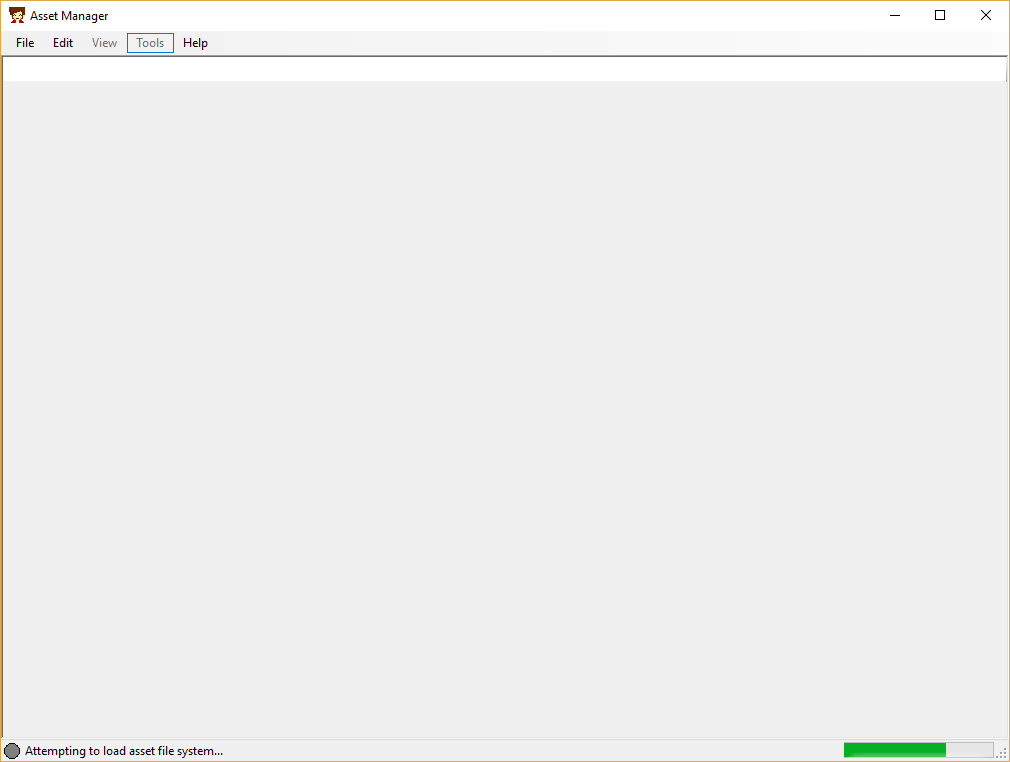The photograph showcases an application window prominently outlined in yellow. At the top of the window, a cartoon character with dark hair is displayed beside the title "Asset Manager" in black text. The window features conventional user interface elements, including the minimize, maximize, and close buttons. Beneath the title, the menu bar lists several options: "File" and "Edit" in black, with "View" and "Tools" grayed out. Despite being inactive, "Tools" is highlighted with a blue box. The "Help" option is also visible.

Below the menu bar, a thin white strip spans the width of the application, transitioning into a gray background that dominates the rest of the window. Noteworthy at the bottom is a gray circle icon followed by the text "Attempting to load asset file system..." A green progress bar, approximately 60% filled, extends towards the right, indicating the current progression of the loading process.